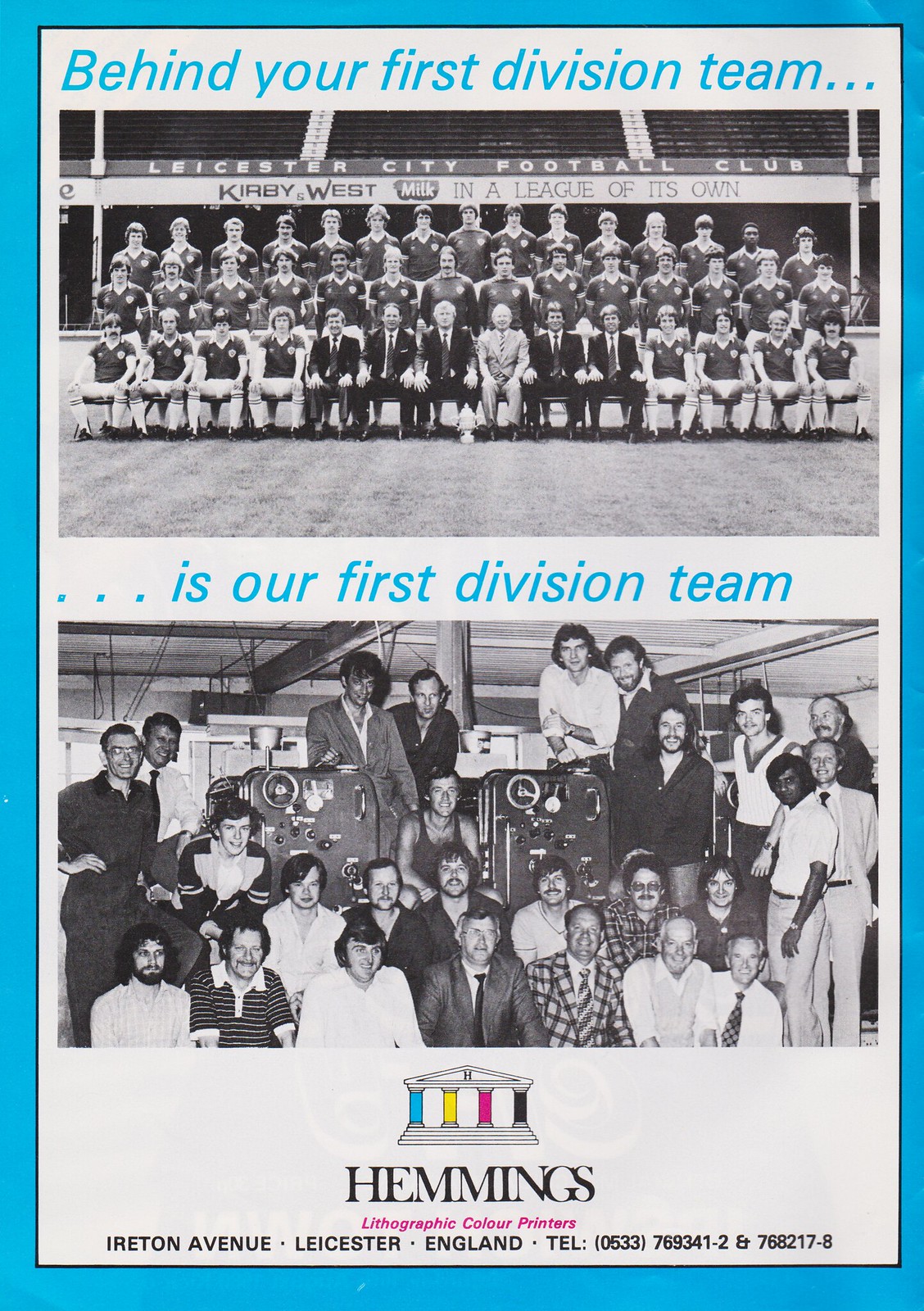The image is a page from a sports paper with an aqua blue border and a slender white rectangular space in the center, bordered in black. At the top of the white space in italicized blue text, it says, "Behind your first division team is our first division team". Below this, there are two black-and-white photographs divided by a white space. The first photo shows a football team seated in three rows, with coaches and possibly other officials in formal attire (shirts, ties, and tuxedos) in the front row. Behind them, text reads: "Leicester City Football Club, Kirby and West Milk, in a league of its own", displayed across the bottom of stadium seats. The second photo depicts a large group of people, also formally dressed, with a man in a notably plaid jacket among them, likely associated with the team. At the bottom of the page, there is a colorful logo resembling a Roman temple with four pillars in blue, yellow, pink, and black. Below the logo, it says, "Hemmings Lithographic Colour Printers, Aylestone Avenue, Leicester, England, Telephone 0633-78934-2 and 78217-8" for contact details.